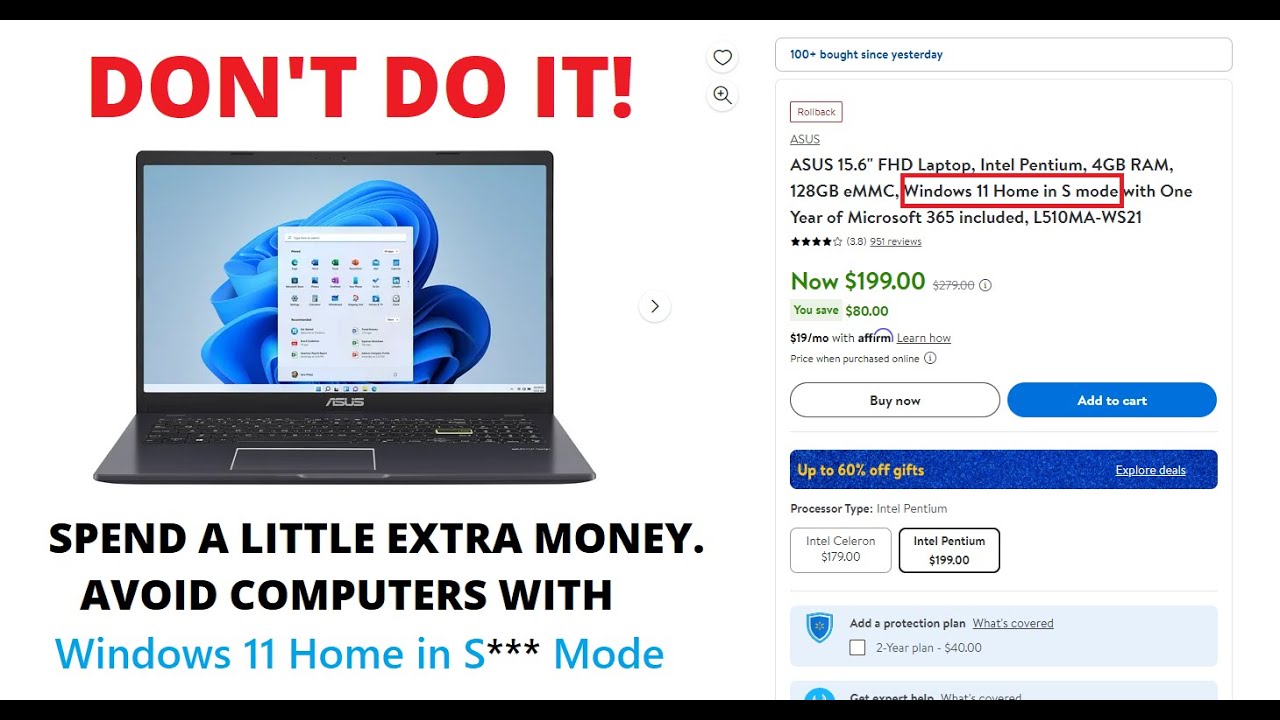**Screenshot of an ASUS Laptop Advertisement on a Website**

The screenshot features a website with a black border both at the top and bottom. On the left-hand side is the focal point: an image of a sleek black ASUS laptop, displaying a gray and blue wallpaper. Prominently, in large red bold font, it cautions, "Don't do it!" Below this, a cautionary note in black font advises, "Spend a little extra money, avoid computers with Windows 11 Home in S*** mode."

In the upper right, various utility icons are visible, including a favorite icon and a zoom icon, accompanied by the text "100+ brought since yesterday." The advertisement details the ASUS 15.6 FHD laptop, specifying key features such as an Intel Pentium processor, 4GB RAM, 128GB eMMC storage, and Windows 11 Home in S mode, with a one-year subscription to Microsoft 365 included (model: L510MA-W321).

The laptop is offered at a reduced price of $199, providing an $80 saving, or available for $19 per month with Affirm financing. Additionally, there's a prompt to "Learn how" regarding the payment options. The purchase options include a "Buy Now" or "Add to Cart" button. Enhanced details about the sale include "Up to 60% off gifts" and further deals to "Explore."

Lastly, there's a specification of processor types with respective prices: an Intel Pentium for $199 and an Intel Celeron for $179. Customers are also given the option to add a protection plan for two years at an additional cost of $40.